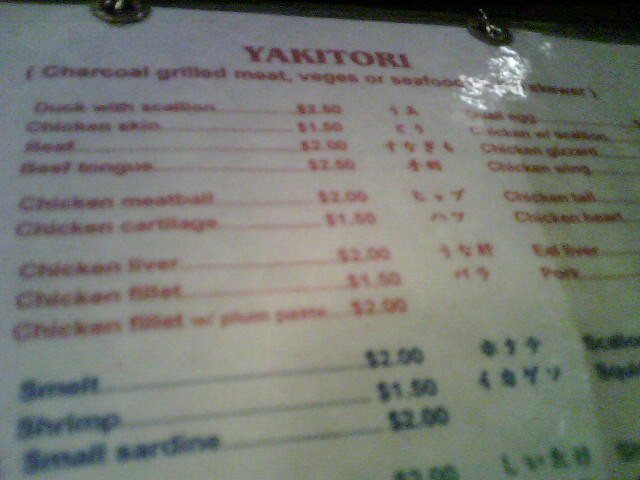This image depicts a detailed menu from a Japanese yakitori restaurant. At the top, the bold red heading "Yakitori" prominently indicates the restaurant's specialty in charcoal-grilled meats, vegetables, and seafood. The menu features a variety of items under different headings distinguishable by color. The meat section, highlighted in red, lists options such as duck with scallions, beef, chicken meatball, chicken cartilage, and chicken liver, with prices ranging from $1.50 to $2.50. Below this, the seafood section is marked in blue and includes choices such as shrimp and sardine, priced at $1.50 and $2.00 respectively. Although the green section's contents remain mostly obscured, part of a price is visible. The menu is designed with items listed on both the left and right sides, and Japanese writing between them, which may either describe the menu items or serve another purpose. The menu is held together with rings at the top and is laminated, as evidenced by the glare on its surface.